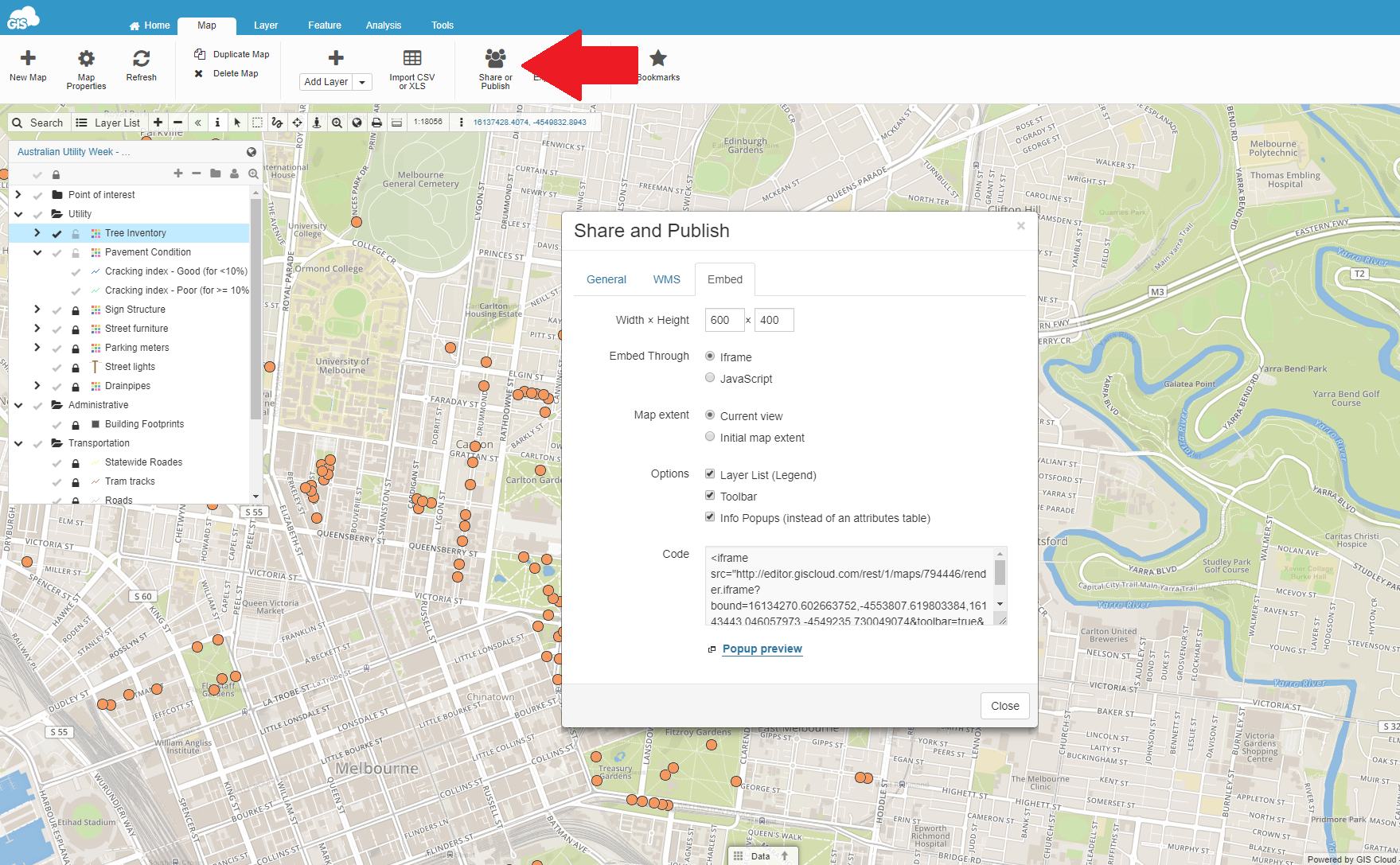The image depicts a detailed Geographic Information System (GIS) interface. At the top, there is a navigation banner with tabs indicating various sections. The tabs include "GIS" with a cloud icon behind it, "Home," "Map" (which is highlighted in black), and "Layer Feature Analysis." Below the navigation banner, the background turns white, showcasing various options in black text: "New Map," "Map Properties," "Refresh," "Duplicate Map," "Delete Map," "Add Layer," "Import CSV or XLS," "Share or Publish" (highlighted by a red arrow pointing towards it), and "Bookmarks" (denoted by a star icon).

The main portion of the interface features a map with multiple orange circles representing different data points. The map includes clearly labeled streets such as Queensbury Street, Swanson Street, Victoria Street, Queens, Victoria Market, Franklin Street, A. Beckett Street, Melbourne, William Street, Bourke Street, and Spencer Street. 

On the left-hand side, there is an open tab with a list of categories. The tab, highlighted in blue, is labeled "Australian Utility Week." Underneath, a series of categories are listed in black text, including "Point of Interest," "Utility," "Tree Inventory" (which is highlighted in blue), "Pavement Condition," "Cracking Index (Good, <10%)," "Cracking Index (Poor, ≥10%)," "Sign Signature," "Street Furniture," "Parking Meters," "Street Lights," "Drain Pipes," "Administrative Buildings," "Footprints," "Transportation," "Statewide Roads," "Tram Tracks," and "Roads."